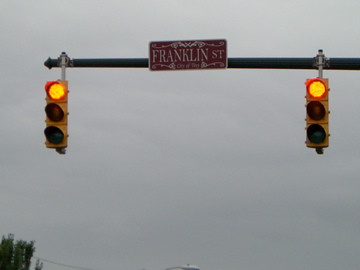The photograph captures a scene dominated by a cloudy, gray sky, creating a somber backdrop. In the lower left-hand corner of the image, partial green treetops emerge, adding a touch of color. A dark gray-to-black horizontal pole extends from the right side, traversing nearly three-quarters of the image. Two yellow traffic lights are suspended from this pole, one on the far left and one on the far right. They both display an illuminated red light, though one appears slightly yellowish. Centrally positioned on the pole is a red street sign, framed by white squiggly borders at the top and bottom, boldly stating "Franklin ST." A wire and possibly a thin white pole, perhaps for a street light, can also be seen faintly near the bottom of the image.